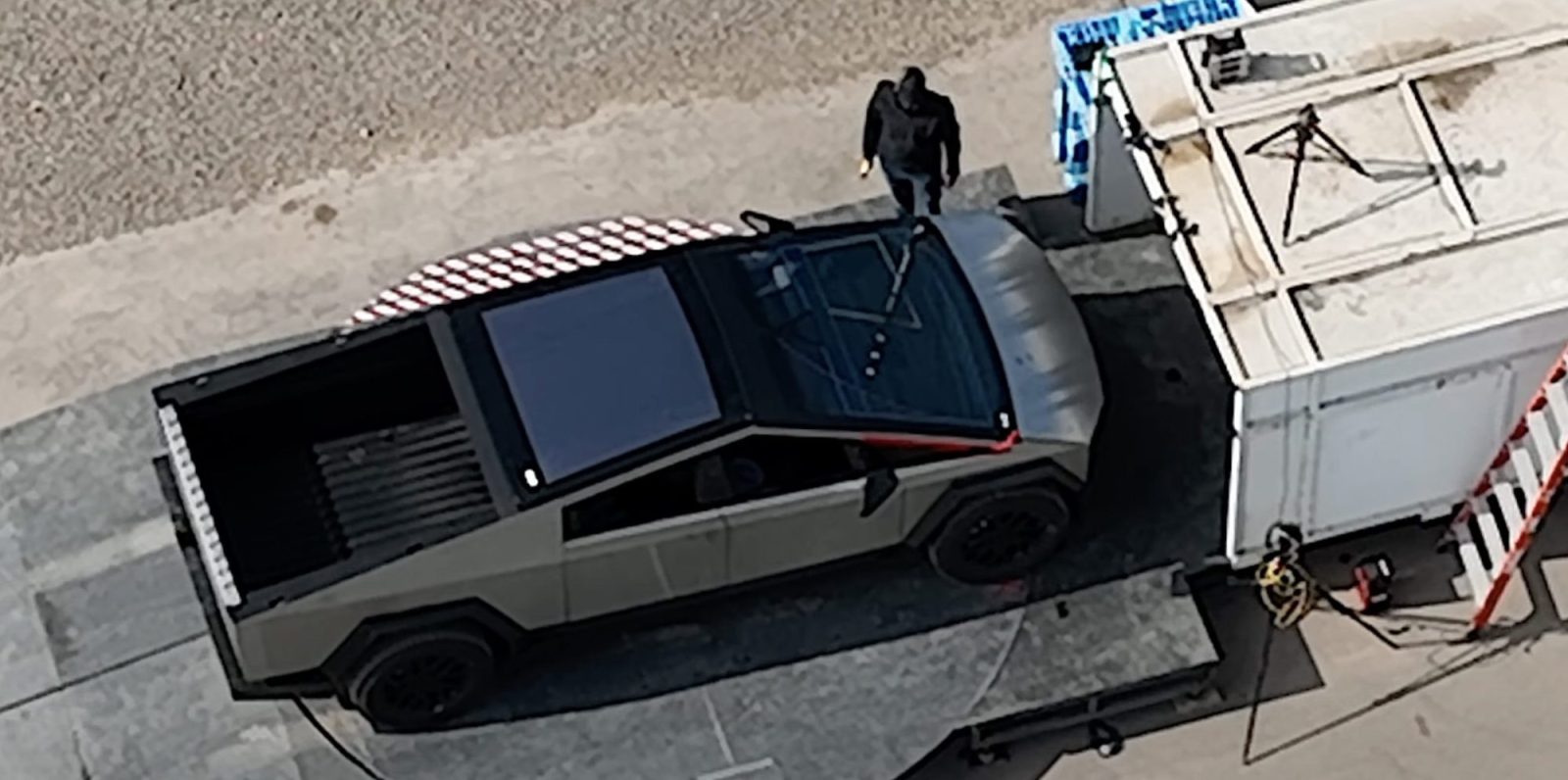An aerial view captures a distinctive scene centered around a blocky, angular vehicle resembling a Tesla Cybertruck, though its precise model is not confirmed. The car is predominantly brown with a black top, potentially featuring either a window or a solar panel. The top-down perspective shows the vehicle being loaded into a large, dull white container or trailer via a black ramp. This container occupies the right side of the frame, perfectly sized for the vehicle. The scene takes place on a concrete lot, characterized by its beige and gray hues. A person dressed entirely in black, possibly including jeans and headwear, stands near the top center of the image, observing the situation. Notably, a ladder with orange sides and silver steps is visible at the bottom right, adding an industrial touch to the overall setting.